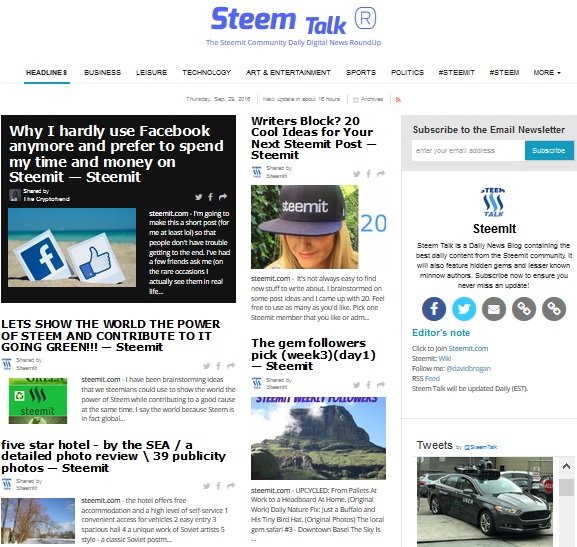**Caption:**

This detailed screenshot showcases a webpage from a community called "Steam Talk." The title "Steam Talk" is prominently displayed in blue with a registered trademark symbol (®) beside it. Below this is a smaller blue tagline, "SEMA Community Daily Digital News Roundup." 

At the top of the page, a black menu bar offers various navigation options: Headlines, Business, Leisure, Technology, Art and Entertainment, Sports, Politics, and more. Notably, hashtags like #steemit and #steam appear, with "steam" explicitly spelled as S-T-E-E-M.

The main content area, though slightly blurry, reveals a divided layout. On the left, a black box contains text, "Why I hardly use Facebook anymore. I prefer to spend my time and money on Steemit." This is accompanied by an image of a blue Facebook icon and a "Like" button buried in the sand on a beach. Adjacent to this, another section titled "Writer's Block: 20 Cool Ideas for Your Next Steemit Post" provides inspiration for content creation.

On the right side, a gray box invites users to subscribe to the email newsletter. It includes an input field and a blue "Subscribe" button. Below this, a call-to-action reads, "Let's show the world the power of Steem and contribute to it going green, Steemit."

Further down, the page features additional articles:
- "Five-Star Hotel by the Sea: A Detailed Photo Review" featuring 39 publicity photos.
- "The Gem Followers Pick: Week Three, Day One," both highlighting the thriving "Steemit" community.

Overall, the page design emphasizes interactivity and the vibrant contributions of its user base.